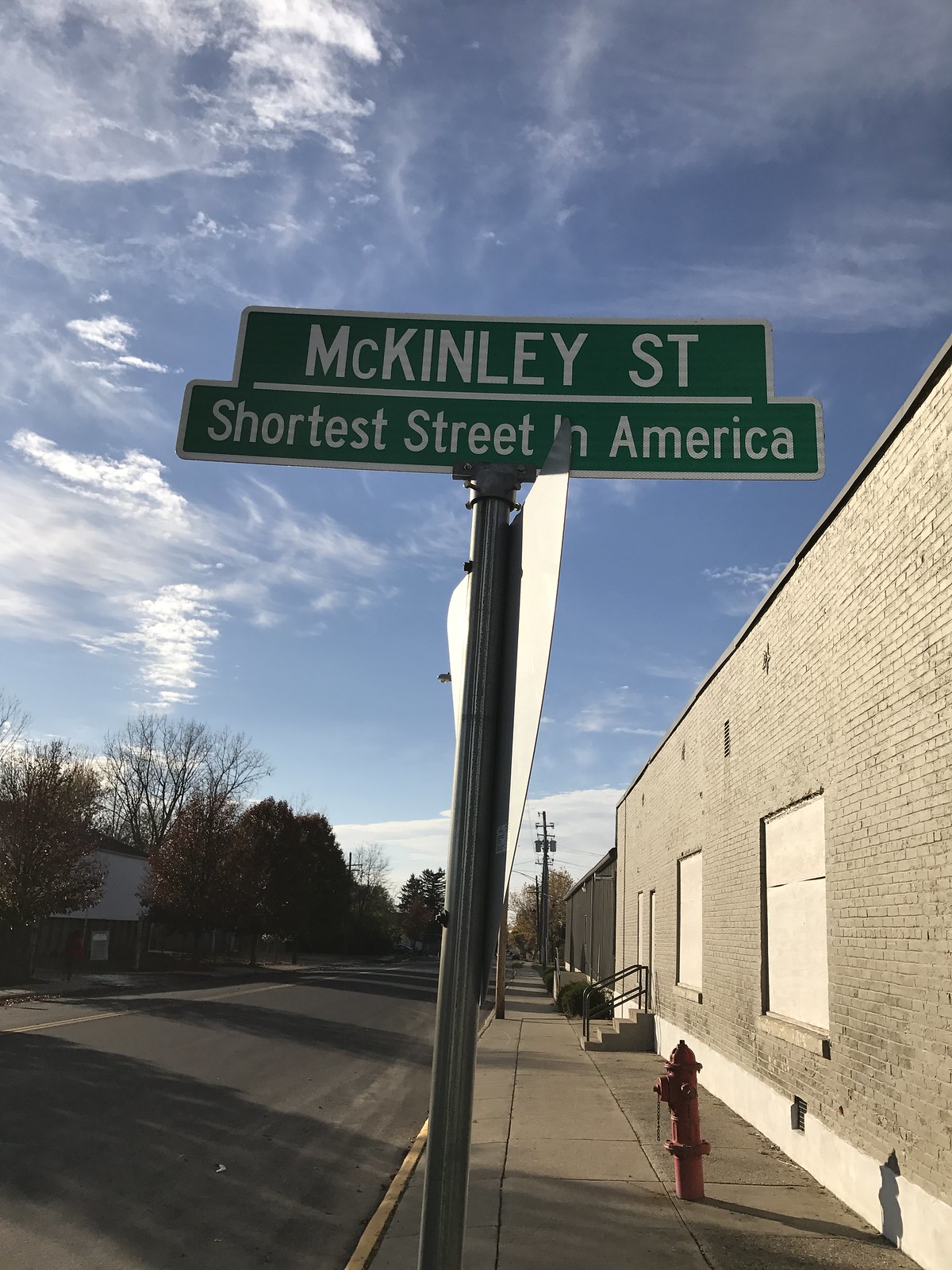This image captures a street scene with the primary focus on a street sign taken from a low angle, looking upward. The sign prominently displays "McKinley Street" with an additional smaller sign beneath it that reads "Shores Street America." In the lower left-hand corner of the image, there is a visible portion of the roadway. The lower right side shows a sidewalk, which runs parallel to the street depicted. Further to the right, a building with closed dock doors is visible, indicating its use for truck loading. The docks are elevated, suggesting they are intended for trucks to back into for loading or unloading. The perspective of the photograph is from the street level, looking down the intersection where the sidewalk and street converge.